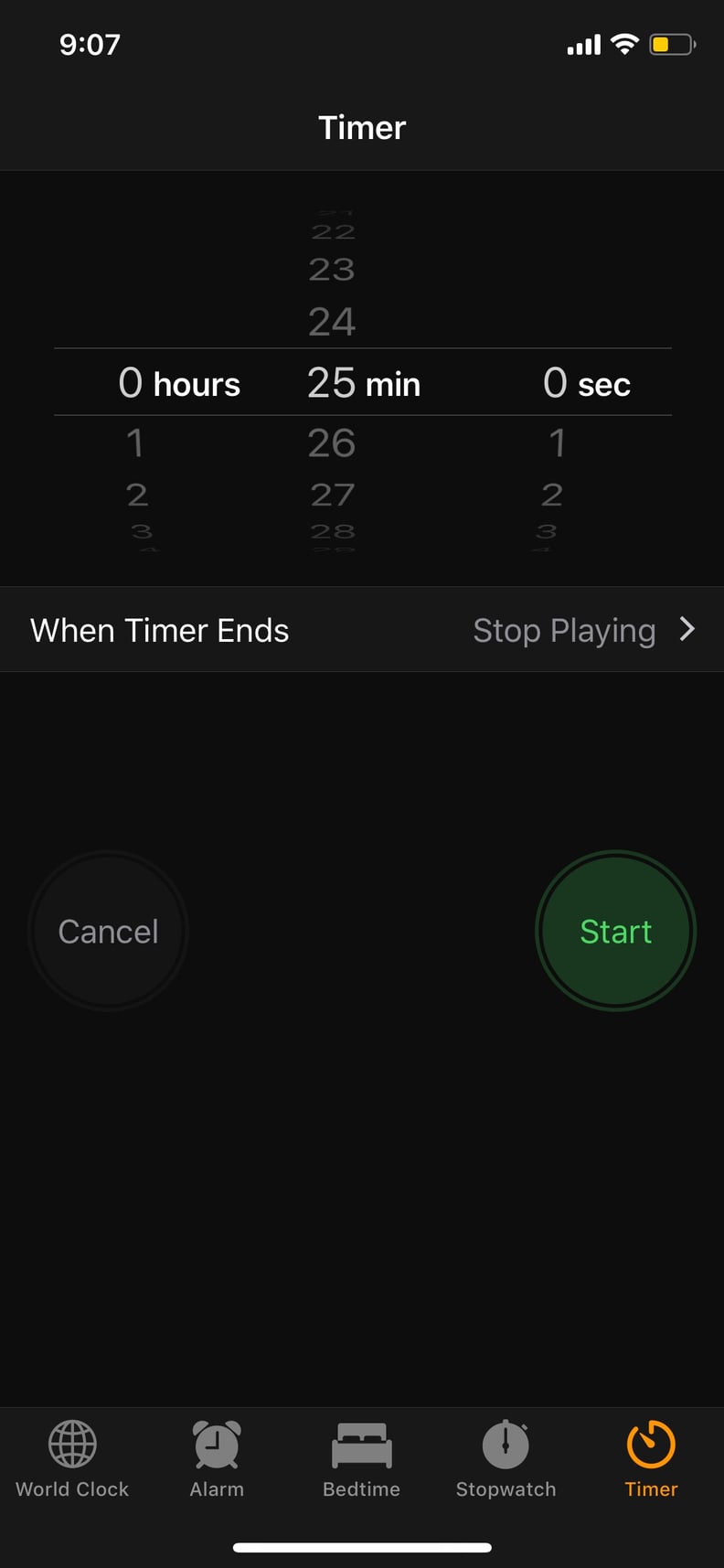This image is a screenshot of the timer screen on an Apple Watch, featuring a minimalist black background. In the upper left corner, the time is displayed as "9:07". The upper right corner includes a signal indicator, a Wi-Fi icon, and the battery percentage. Dominating the center of the screen, the word "Timer" is prominently displayed in white, followed by the timer settings showing zero hours, 25 minutes, and zero seconds.

Beneath the timer settings, there is a message stating, "When Timer Ends: Stop Playing." Below this are two touchable options: a white "Cancel" button on the left and a green "Start" button on the right. Along the bottom, five icons are aligned in a row, all in gray except for one. These icons include a sphere labeled "World Clock," an alarm clock labeled "Alarm," a bed labeled "Bedtime," a stopwatch labeled "Stopwatch," and, highlighted in orange, a timer labeled "Timer."